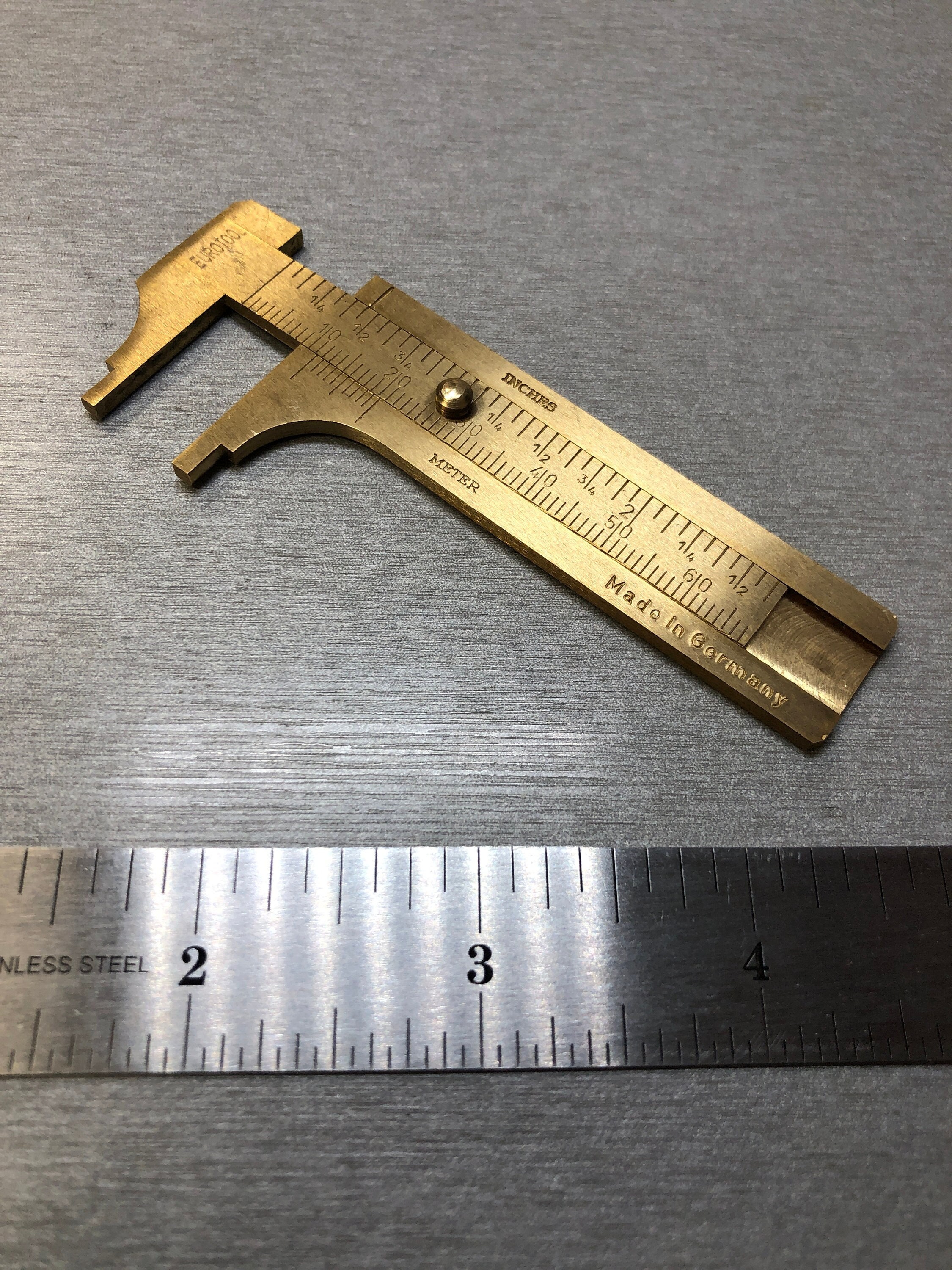This is a detailed color photograph of measuring equipment laid out on a metallic gray background, which gives off a slight reflection. At the bottom of the image, there is a stainless steel ruler displaying the 2, 3, and 4-inch marks, as well as centimeter measurements. Above the stainless steel ruler, there is a brass-colored caliper inscribed with "Made in Germany." This caliper resembles a tool with a clamp-like feature at the top and includes an adjustable sliding component that allows for precise measurements by pinching an object. The caliper also has markings for inches and meters. Both tools are positioned parallel to each other on the gray tabletop surface, with no people, animals, buildings, or vehicles visible in the image.